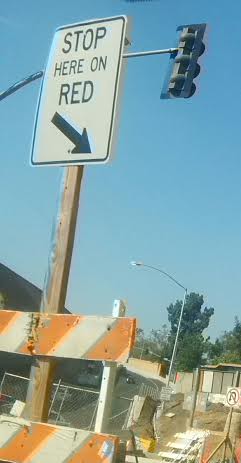A close-up, daytime photograph captures a busy construction site under a clear blue sky, framed by scattered distant trees and streetlights. In the upper portion of the image, the back of a black traffic light peeks in, while to the left an orange and white diagonal-striped construction guardrail stands prominently. Attached to this guardrail is a white metal sign with bold black lettering directing, “STOP HERE ON RED,” accompanied by a downward-right arrow. Below this, another small sign forbids U-turns. The scene is a blend of active construction elements and everyday traffic controls.